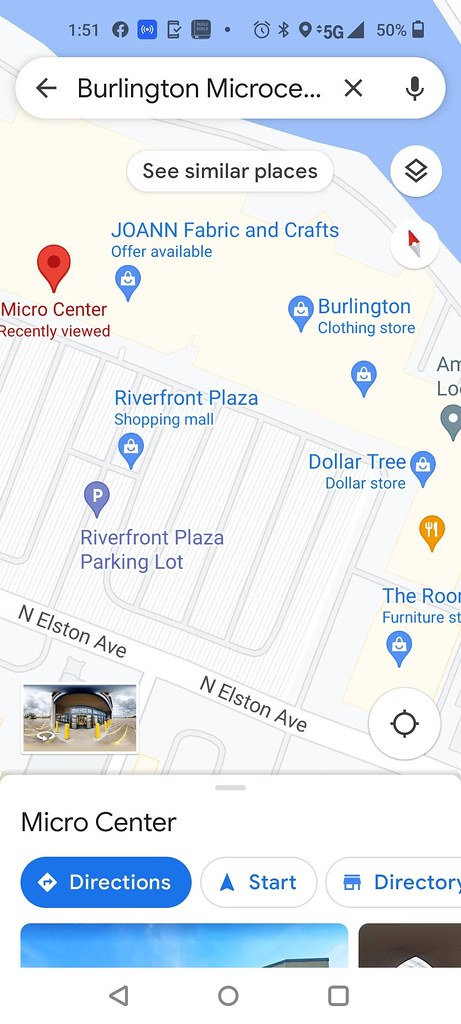This image is a detailed rectangular portrait screenshot taken from a cell phone displaying a navigation map. The image has a vertical orientation, approximately three times as high as it is wide. There is no border shown around the image.

The upper portion of the image is dominated by the map which extends through the header area. The top section of the map features a body of water, possibly a sea or lake, in a medium blue color, which angles from the upper left corner to about 40% down on the right.

Across this blue water background, the top strip of icons is visible. From left to right, the strip displays the following:
1. The time: "1:51".
2. The Facebook icon.
3. Three additional icons.
4. A small black dot.
5. The clock (alarm) icon.
6. A few more icons.
7. The indicator "5G".
8. A right triangle ascending icon indicating signal strength.
9. The percentage "50%" showing battery level.
10. A vertical battery icon, approximately 50% full.

Below this icon strip is the search field, which is a long white rectangle with rounded corners. It features:
- A short arrow pointing left.
- The partially obscured search term "Burlington micro sit, M-I-C-R-O-C-E...".
- A gray 'X' on the right side.
- A microphone icon signifying voice search.

Directly beneath the main search bar, there is a smaller, similar white rectangle with rounded corners that reads "See similar places". To its right, there is a white circle featuring two stacked diamond icons.

The map, which occupies most of the image, has a white background with roads and various landmarks highlighted. The upper left corner displays a water body with roads running parallel to the shore. The layout of the area is somewhat grid-like, but angled such that it descends approximately 30 degrees from left to right. There are numerous vertical roads forming the grid, with fewer horizontal roads.

Highlighted locations on the map include:
1. Micro Center - Located towards the left side of the image, slightly north of center, marked by an upside-down teardrop pin in red. It is labeled "Micro Center" with "Recently Viewed" beneath it.
2. Joanne Fabric and Crafts - Situated to the right of Micro Center, marked by a medium blue pin.
3. Burlington Clothing Store - Found on the right side, parallel to the previous locations, also marked with a pin.
4. Riverfront Plaza Shopping Mall - Positioned left of center within the road layout, marked with a pin.
5. Dollar Tree - Marked with a pin on the right side within the road grid.

In the lower-left corner, there is a photograph of what appears to be the Micro Center building, surrounded by a large parking lot. 

The bottom 20-25% of the image, just below the map, is dedicated to navigation options for Micro Center:
- The name "Micro Center" in the upper left.
- A long blue button labeled "Directions" in white text.
- Two white buttons with blue fonts on the right side: one labeled "Start" and the other labeled "Directory".